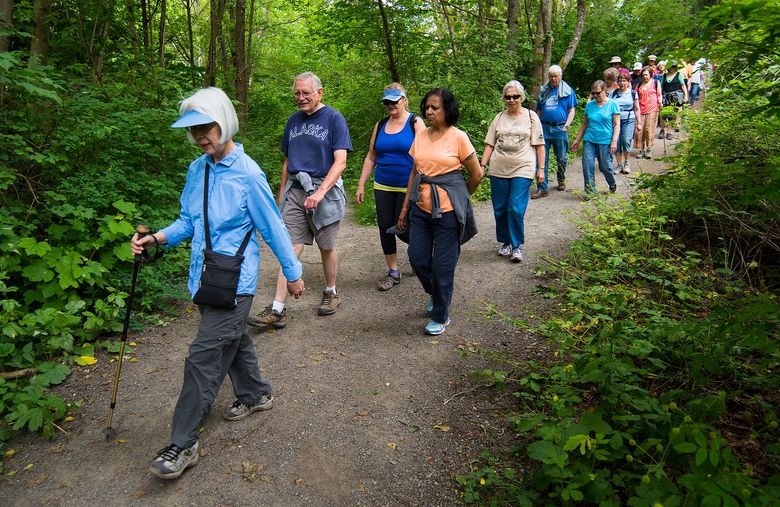In this vibrant and sunny photograph, a large group of hikers is seen making their way down a dirt gravel path that winds diagonally through a lush, green forest. The trail, framed by trees and verdant undergrowth on either side, appears to be part of a park. Leading the group is an older woman, likely in her 60s or 70s, wearing a blue long-sleeve shirt, dark gray pants, sneakers, and a blue visor. She carries a walking stick and has a pouch strapped to her front. Following her are several other hikers, including a man in a blue shirt emblazoned with "Alaska" and gray khaki shorts, and a woman dressed in an orange shirt. The hikers, mostly in their late 40s to 70s, are clad in a mix of shorts, pants, and various types of hiking gear. While some carry walking sticks, many do not, suggesting a leisurely group hike rather than a competitive race. The scenery, combined with the cheerful expressions of the hikers, indicates that it is a pleasant and enjoyable day to be out in nature.